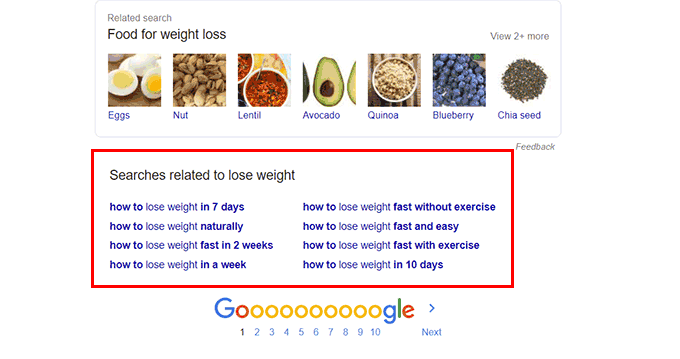This image is a screenshot of a Google search on a smartphone. At the top of the screenshot, it displays the heading "Related search" followed by the phrase "food for late loss" in black text, likely a typo intended to refer to weight loss. Below this heading are seven small boxes, each with a picture and the name of a corresponding food item. The food items listed are:

1. Eggs
2. Nuts
3. Lentils
4. Avocados
5. Quinoa
6. Blueberries
7. Chia seeds

Each food item includes an associated picture. Underneath these boxes, there is a prominent red rectangular box containing the text "Searches related to lose weight," followed by eight clickable Google search suggestions. These suggestions are:

1. How to lose weight in seven days
2. How to lose weight fast without exercise
3. How to lose weight naturally
4. How to lose weight fast and easy
5. How to lose weight fast in two weeks
6. How to lose weight fast with exercise
7. How to lose weight in a week
8. How to lose weight in ten days

At the bottom of the screenshot, there is a Google logo with numbers one through ten below it, along with a "Next" button, indicating pagination for further search results. To the right, there is a grey "Feedback" button at the top, providing an option for users to give feedback on the search results.